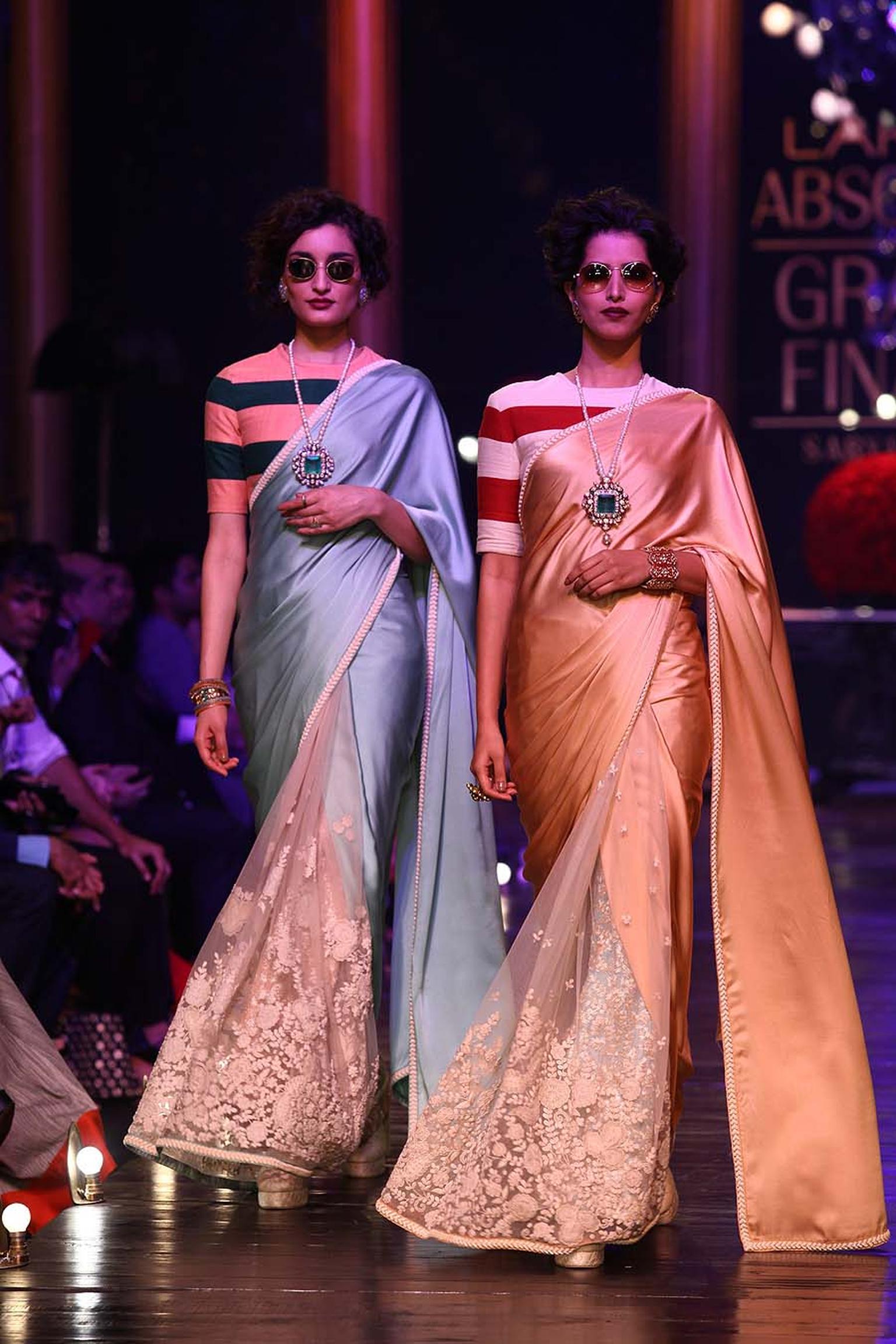In this photograph, two women are walking down a runway, modeling in strikingly coordinated, Indian-style saris draped over their shoulders. Their outfits consist of vibrant, striped half-sleeved shirts underneath: the woman on the left wearing a salmon and navy pattern, and the woman on the right in white and red stripes, both matching the color of their saris. They each sport long, exquisite necklaces embellished with large blue gemstones and wear identical sunglasses that complement their curly brown hair and darker skin. Enhancing their sophisticated look, they also adorn luxurious bracelets and rings. The subdued, dark lighting casts a mysterious ambiance over the scene, and a blurry audience can be seen in the background along with partially visible text. The models' posed, synchronized steps, with their left arms resting across their stomachs and right arms hanging down, highlight their seamless presentation.